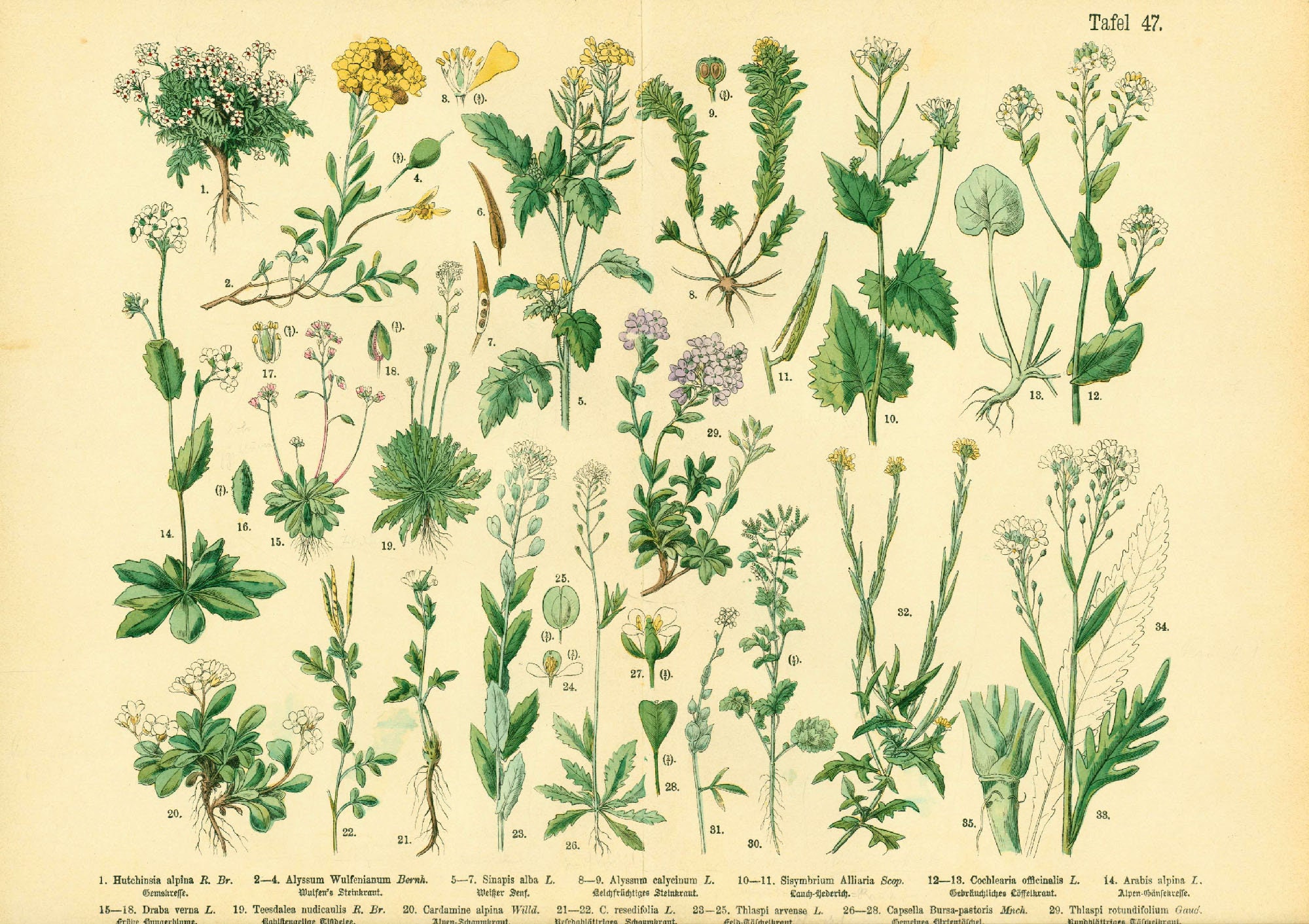This up-close image is a detailed botanical illustration of approximately 35 different types of herbaceous plants, depicted on an aged parchment-style background typical of old school textbooks. Each plant is uniquely numbered and referenced in a corresponding legend at the bottom of the page that lists the genus and species, although the text is too small to read clearly. The illustration showcases various plant structures, including a variety of leaf shapes, from short and stout to long and spindly, and features an array of flowers, some with extra petals and others resembling dandelions with elongated leaves and tiny flower petals. The plants are primarily rendered in shades of green, with accents of brown, yellow, and white. Notably, the top right corner bears the black-inked inscription "Tafel 47," indicating its position within a larger collection.